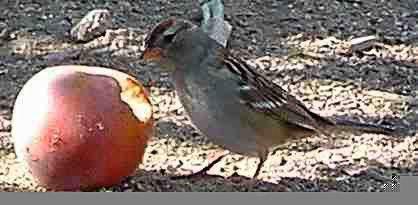In this image, a small, gray-colored bird is captured in the center, actively pecking at a red apple. The bird exhibits a gray chest, light brown wings adorned with white specks, and a patch of orange on top of its head. It has a short orange beak and black eyes. The bird is positioned with one foot forward towards the apple and the other almost straight down, facing left with its long tail extending towards the right. The apple, which shows signs of having been pecked, reveals a light yellow, slightly browning interior and reflects white light off its dirty red exterior. Surrounding the scene is a ground composed of light brown and gray dirt, interspersed with small rocks, including a notably light gray, rectangular one behind the bird's head. The background features shadows at the top and brighter lighting at the bottom. A gray line runs across the bottom of the image, bulging slightly before exiting to the right, adding a subtle boundary to the earthy, natural setting.